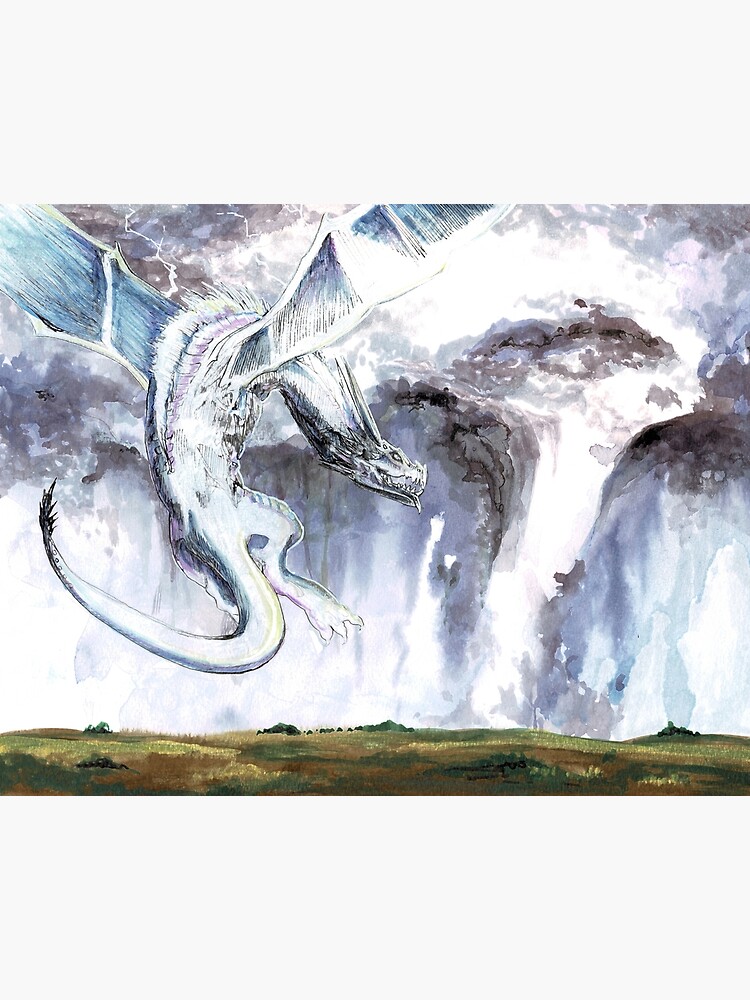The watercolor painting depicts a majestic, predominantly white and black dragon with blue accents on its wings, soaring through the sky. The dragon's wings are spread wide, showcasing intricate blue with black stripes, while its long tail trails behind. The dragon's head, which resembles a large lizard, is angled downward, revealing sharp fangs protruding from its mouth and horns atop its head, suggesting impending anger. Beneath the dragon, the earth is illustrated with a lush, undulating grassland in various shades of green, yellow, and tan, giving a vibrant contrast to the splotchy, drippy blue hues of the sky above. A striking element in the background is a swirling tornado in white, dark gray, and black, larger at the top and tapering toward the ground, adding a sense of impending drama to the scene. The overall effect creates a dynamic composition, emphasizing the dragon in flight over a vivid, watercolor landscape.